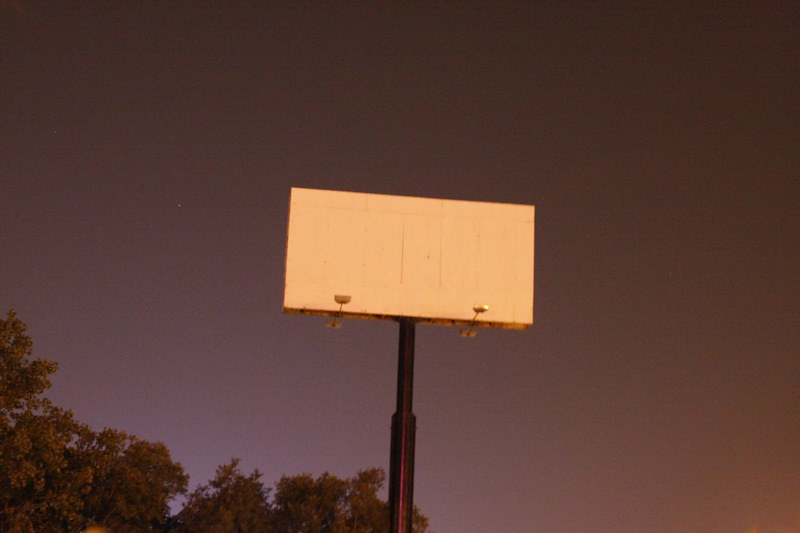This photograph captures an evening scene of an empty billboard viewed from street level. The black metal pole, thick and sturdy, supports the billboard, which appears some distance away. Two lights extend outward from the billboard's lower edge, though they remain unlit, suggesting twilight is just settling in. The billboard itself is stripped of any advertisements, revealing a plain surface made up of white panels. A noticeable vertical crease or crack runs through the center of the billboard, adding an element of imperfection to the otherwise blank canvas.

The sky in the background is a deepening shade of blue, bordering on black but not yet fully transitioned into night. A few stars have already appeared, twinkling faintly. To the left of the frame, the tops of trees are visible, their silhouettes adding a touch of nature to the urban landscape.